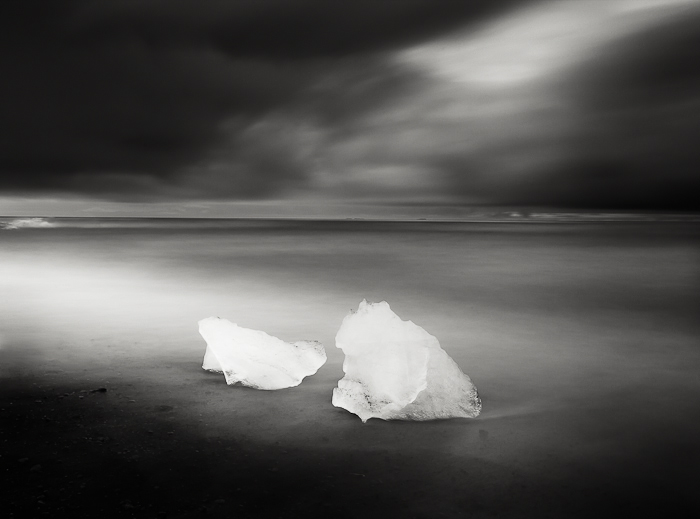The image depicts a surreal and ominous scene, blending elements of the natural and the otherworldly. Central to the composition are two bright white, crystal-like structures reminiscent of seashells, standing out starkly against a predominantly gray and black backdrop. The landscape is flat and expansive, evoking the surface of another planet. The ground is mirror-smooth, reflecting the turbulent, cloudy sky above, which hints at an impending storm. The photograph's square frame encapsulates a horizon line that hints at distant, indiscernible features, possibly water, with hints of white caps breaking the uniform darkness. The overall monochromatic palette, with varying shades of gray, enhances the otherworldly and serene, yet foreboding, atmosphere.